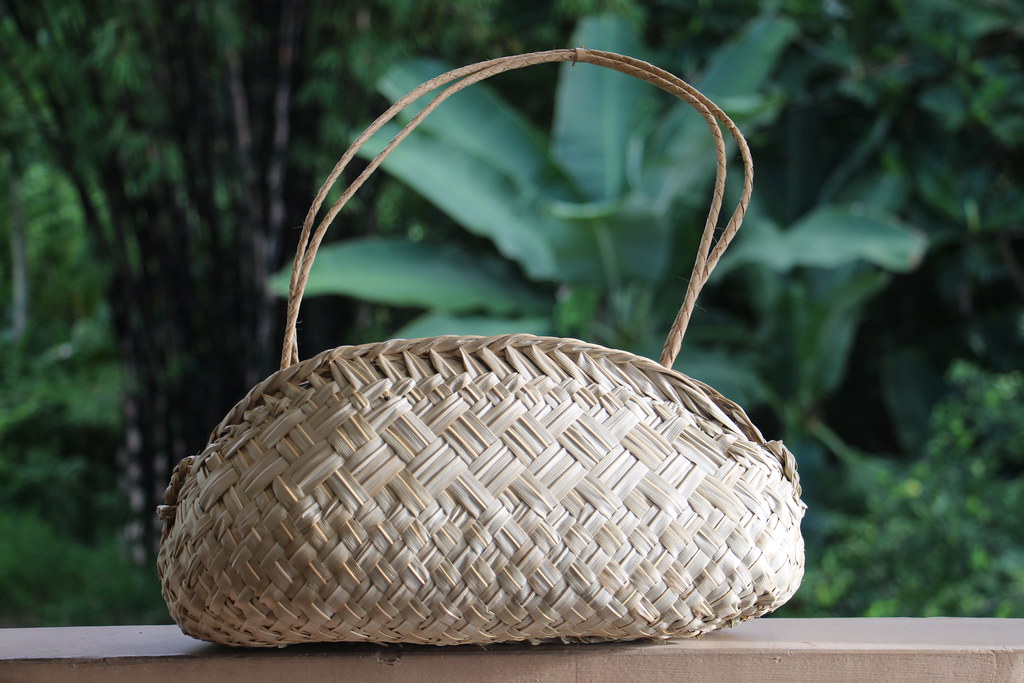This detailed color photograph features a woven basket situated prominently on a cement ledge. The basket, which appears to be made from thin, light brown, plant-based materials like reeds or wicker, showcases intricate diagonal crisscross patterns that mesh together, creating a textured surface. The thin handle, also woven from similar materials, adds to its delicate appearance. Illuminated by sunlight from the right, the basket stands out against its natural backdrop. The background, though slightly blurred, is lush with various shades of green vegetation, including large, distinctive banana leaves and possibly bamboo stalks, contributing to a serene, natural ambiance. There are no people or visible signatures or dates in the image, allowing the focus to remain solely on the basket and its verdant surroundings.